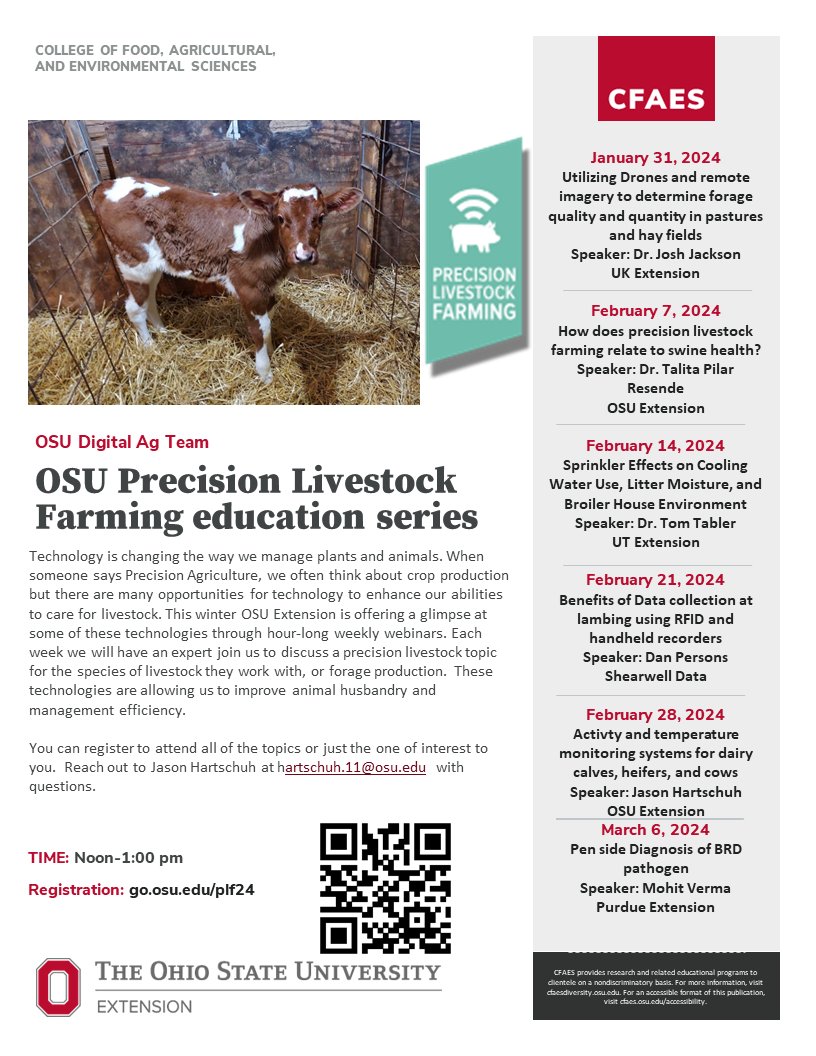This informational flyer from the Ohio State University's Extension, specifically from the College of Food, Agricultural, and Environmental Sciences, details their Precision Livestock Farming Education Series. At the top left, a young cow stands on hay inside a fenced enclosure, emphasizing the focus on livestock. Adjacent to the cow's picture is an illustration of a white pig with Wi-Fi symbol-like curves, representing "Precision Livestock Farming."

The text introduces the OSU Digital AG Team and highlights the technological advancements in managing both plants and animals. The flyer invites the public to join weekly webinars from noon to 1 p.m., where experts will discuss various precision livestock topics, from crop production to animal husbandry. Registration details are provided through a URL (go.osu.edu/plf24) and a QR code, with contact information for Jason Hartschuh (hartschuh.11@osu.edu) for further inquiries.

The right side of the flyer lists the webinar dates and topics: 
- January 31, 2024: Utilizing Drones and Remote Imagery to Determine Forage Quality and Quantity in Pastures and Hayfields, with Dr. Josh Jackson.
- February 7, 2024: How Precision Livestock Farming Relates to Swine Health.
- February 14, 2024: Sprinkler Effects on Cooling Water Use, Litter Moisture, and Broiler House Environment.
- February 21, 2024: Benefits of Data Collection at Lambing Using RFID and Handheld Recorders.
- February 28, 2024: Activity and Temperature Monitoring for Dairy Calves, Heifers, and Sows.
- March 6, 2024: Penside Diagnosis of BRD Pathogen.

At the bottom, within a small, unreadable black section, lies additional fine print.